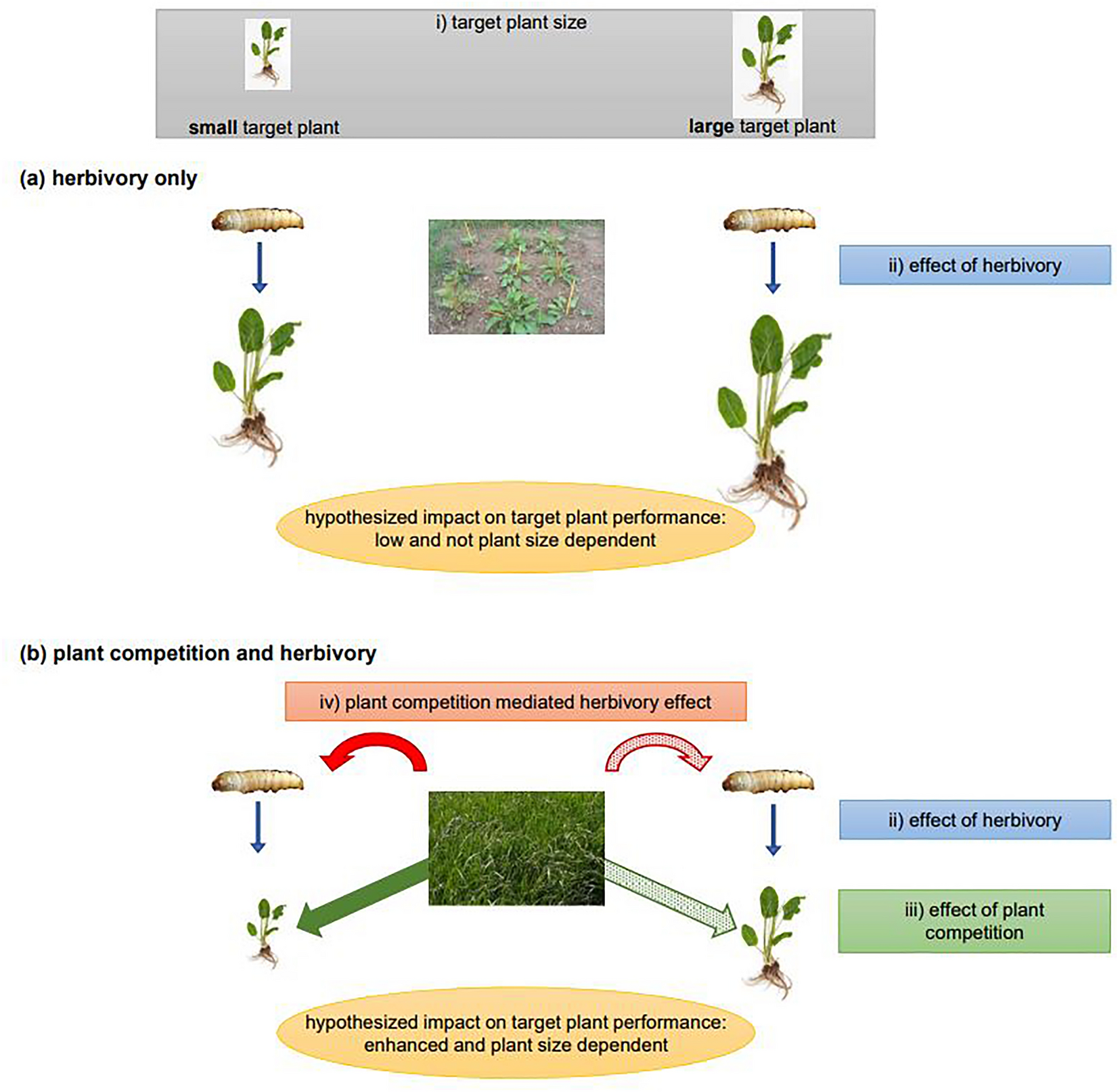This diagram, likely from a textbook or scientific magazine, illustrates the impact of herbivory and plant competition on target plants. At the top, a gray banner labeled "Target Plant Size" divides the diagram into two sections: one side showing a "Small Target Plant" and the other a "Large Target Plant." Below this, the section titled "Herbivory Only" features a small plant with a bug (possibly a snail or slug) near it. Adjacent to this is another plant with the same type of bug. This part of the diagram includes a blue box labeled "Effect of Herbivory" and a yellow oval stating "Hypothesized Impact on Target Plant Performance: Low and Not Plant Size Dependent." 

Beneath this, the section titled "Plant Competition and Herbivory" includes a pink-peach banner reading "Plant Competition Mediated Herbivory Effect." Here, illustrations show bugs with smaller plants and patches of grass pointing to other plants with identical bugs. Adjacent text frames the details: a blue box states the "Effect of Herbivory," an orange box indicates the "Effect of Plant Competition," and another yellow oval explains the "Hypothesized Impact on Target Plant Performance: Enhanced and Plant Size Dependent." Visual elements such as red arrows point to the bugs, blue arrows direct attention to the plants, and a strip of green grass runs through the center, all set against a white background.